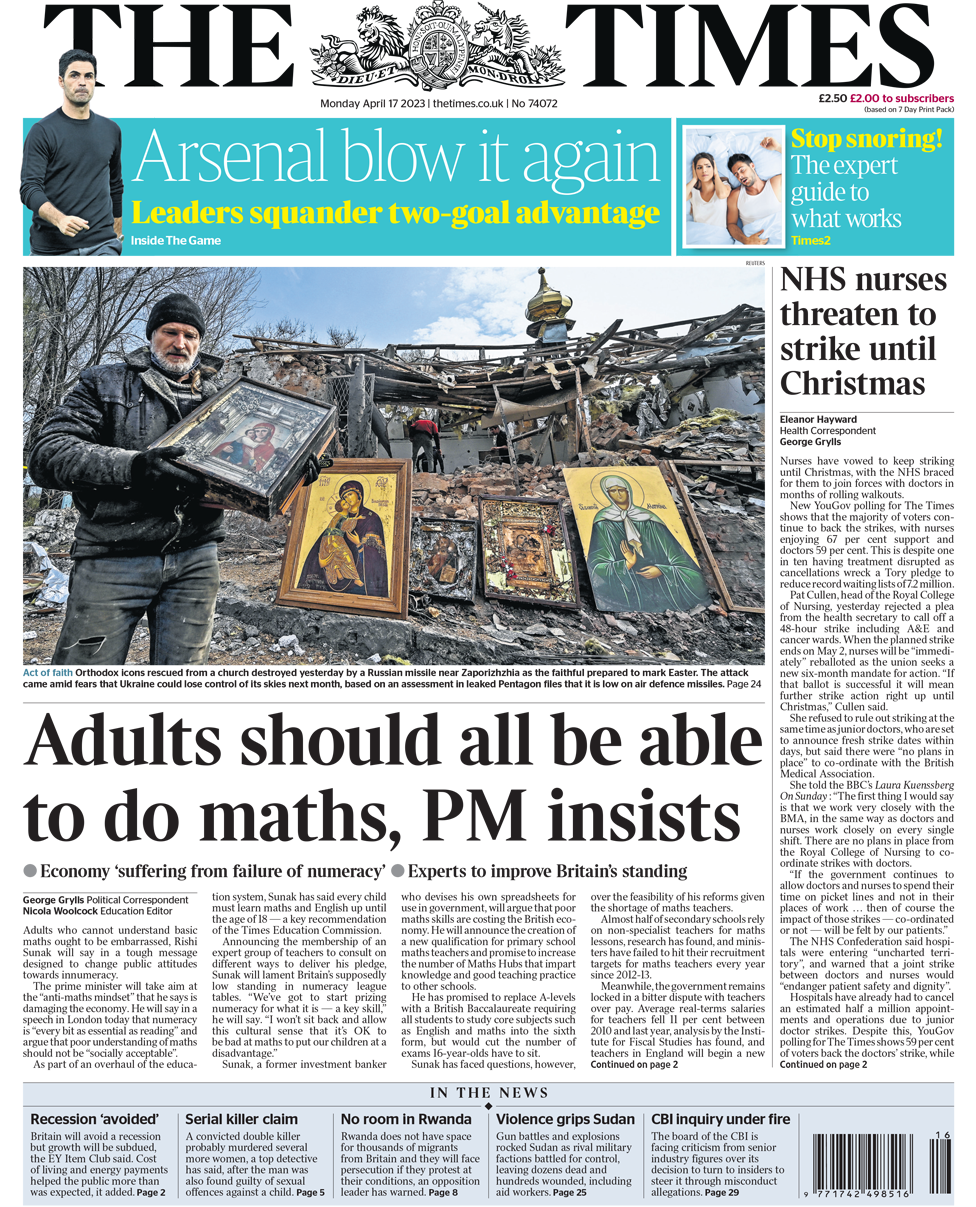**The Times - Monday, April 17th, 2023**

**Arsenal blow it again: Leader squanders two-goal advantage**

Screenshot of a newspaper page from "The Times" website featuring intricate company insignia, including a lion and a unicorn surrounding a crest with Latin text and ornamental designs. The date and website URL "thetimes.co.uk-74072" are displayed below the crest, with pricing details stating the newspaper costs £2.50, with a reduced price of £2 for subscribers on a seven-day print pack basis.

A prominent blue banner headlines, "Arsenal blow it again: Leader squanders two-goal advantage," accompanied by an image of an Arsenal player on the left side to emphasize the story. To the right, an advertisement in blue states, "Stop snoring: The expert guide to what works," featuring a couple in bed.

The main content area features a large rectangular image on the left of a man standing before a burned building, holding a religious painting, with more artwork visible behind him. Below this image is a caption providing further context. A bold headline beneath reads, "Adults should be able to do maths, PM insists."

On the right side, a smaller introduction to an article states, "NHS nurses threatened to strike until Christmas." At the bottom, a blue banner titled "In the news" lists several smaller news headlines.